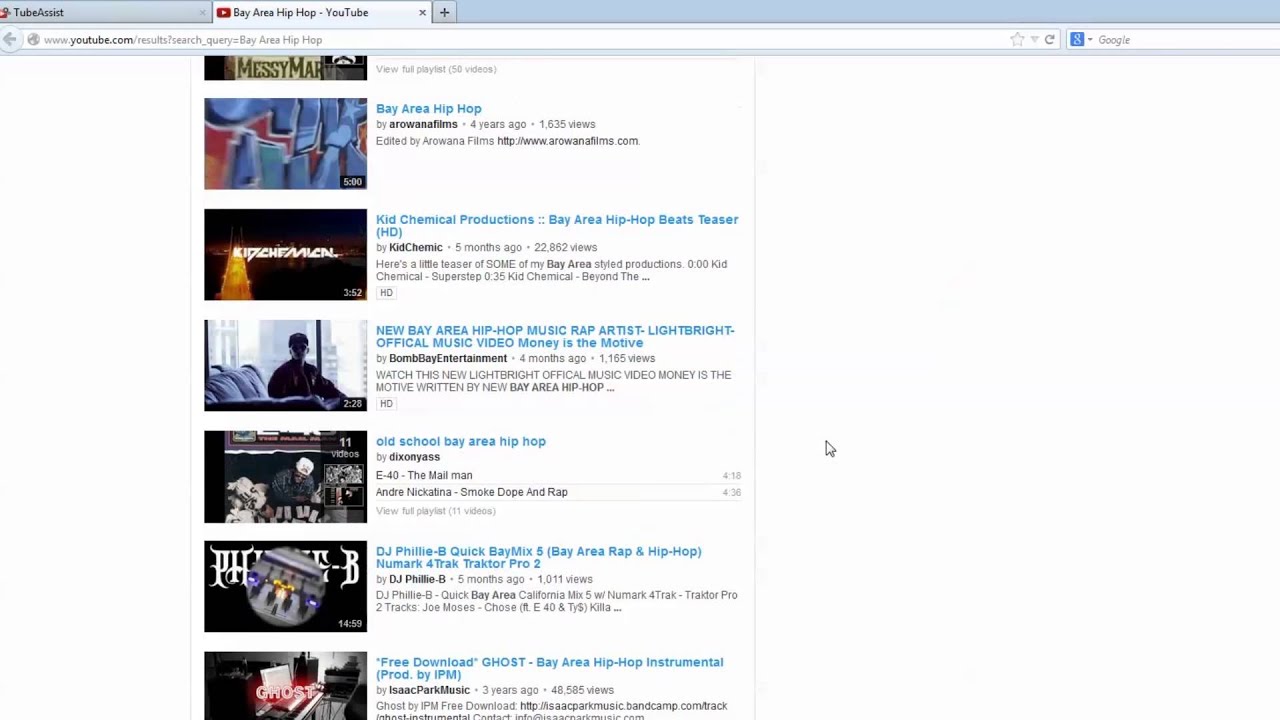This image captures a YouTube search results page for "Bay Area Hip Hop," showcasing a series of video thumbnails and titles organized vertically. Each video entry displays critical details such as the title, channel name, view count, and video duration, adhering to YouTube's standard layout with a white background and black text, complemented by vibrant thumbnails. Prominent videos on the page include "Bay Area Hip Hop" by Arowana Films, "Bay Area Hip Hop Beats Teaser" from Kid Chemical Productions, and "New Bay Area Hip Hop Music Rap Artist Light Bright Official Music Video Money Is The Motive," the latter evidently highlighted by a plugin labeled Tube Assist. This plugin suggests a curated or assisted search experience. The image underscores the user's interest in Bay Area Hip Hop, featuring a mix of old-school and contemporary influences, and likely represents their intention to explore, download, or listen to these tracks.